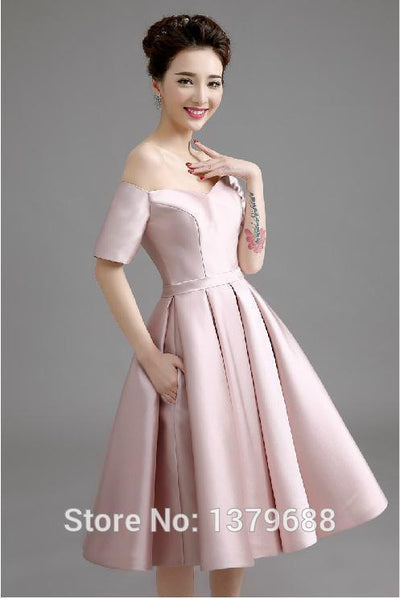This photograph features an Asian woman with dark brown hair styled in an elegant bun, accentuated by a silver needle-like hairstick. She is captured on a gray background, wearing a light pink, metallic-looking off-the-shoulder dress with short sleeves that features vertical pleats and pockets. The woman is smiling directly at the camera, showing her top row of teeth, with flat-shaped eyebrows adding to her gentle expression. Her left hand, adorned with red nail polish, is raised to touch her collarbone area, and a tattoo resembling an upside-down plant with a pinkish flower is visible just above her elbow. Her right hand is partly tucked into the pocket of her dress, showcasing the practical yet chic design of her attire. At the bottom of the image, white text reads "store number: 1379688," indicating a retail reference or catalog number.